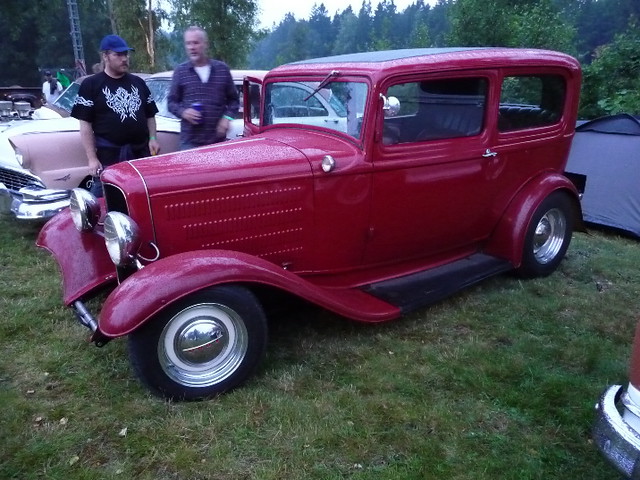This photograph captures a vibrant scene at an antique car show set on a grassy field, with several vintage vehicles and people dispersed in the background against a backdrop of trees. Prominently featured in the foreground is a pristine red early-1900s style car, resembling a Model T or Model A. This meticulously maintained vehicle boasts several distinctive features including a curved fender, two round headlights, and shiny metal hubcaps with painted white rims. It has a small windshield typical of vintage cars, a single windshield wiper on the roof, and a small rear-view mirror on the driver's side. The back window appears to be rolled down or removed, adding to its classic appeal.

Flanking the car, two men appear to be engaged in conversation. The older man, with gray hair, is dressed in a plaid shirt over a white t-shirt and seems to be holding an object, possibly a beverage. Beside him stands a younger man in a blue baseball cap and a black t-shirt with white print. In the background, a glimpse of a pink car and numerous other vintage cars contribute to the nostalgic atmosphere of the show.